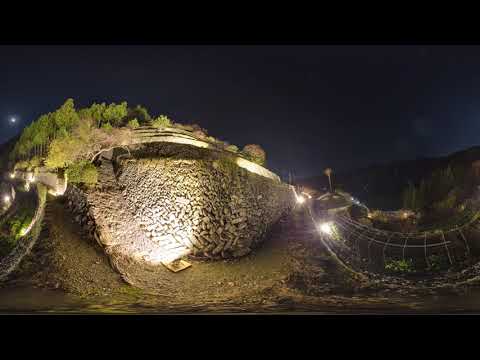This image captures an outdoor nighttime scene dominated by a rugged, rocky hill. The dark sky in the background accentuates the distant presence of the moon just above the hill, which is more of a small, rocky formation. The side of this rocky hill features a series of aligned, retaining rocks. A pathway wrapped around the hill climbs up its side, edged with steps in certain parts. The left-hand side of the image is occupied significantly—about 40%— by this intricate rock formation.

Trees and green brush sparsely dot the top of the hill, adding a touch of life to the otherwise harsh landscape. A small bridge can be seen extending from the top of the formation, leading into the depths of the right-hand side of the image. Beneath the rock, a semicircular patch of brown dirt catches the eye. The right-hand side in the distance features a silhouette of hills, barely discernible against the black sky.

The central part of the image is visibly brightened by artificial lights, causing a glare that washes over the rock’s surface, casting sharp contrasts and shadows. In the foreground, a curious white strip snakes its way across, resembling an earthworm. Although some may find the scene dark and dreary, the detailed interplay of natural and man-made elements provides a complex, multifaceted visual.